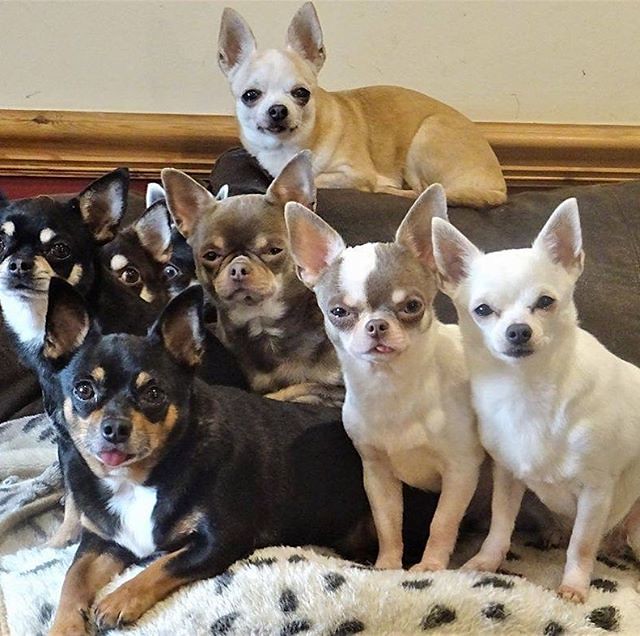This charming photograph captures eight adorable chihuahua puppies snuggled together on a bed inside a cozy bedroom. The backdrop of the image is a light gray wall, partially hidden by a light brown wooden part of the bed frame. The lower half displays a sofa or bed draped with a fluffy white blanket adorned with dalmatian-like black polka dots and a large brown pillow.

In the foreground, the chihuahuas are grouped closely together, all seemingly looking directly at the camera. Among them, four have predominantly black fur with white patches on their chests, and some exhibit brown hues on their feet and around their eyebrows. Two of the puppies are mostly white; one has a bit of black on its face and looks particularly sleepy, sitting on its back paws with its front paws extended. Another chihuahua, sitting atop the brown pillow, is mostly light brown with a white face. Finally, a larger, perhaps matronly chihuahua, stands out with black fur, brown around her eyes, and white along her chest and under her eyes.

The overall scene exudes warmth and coziness, accentuated by the innocent and endearing expressions of the chihuahuas, making for an utterly heartwarming and cute snapshot.